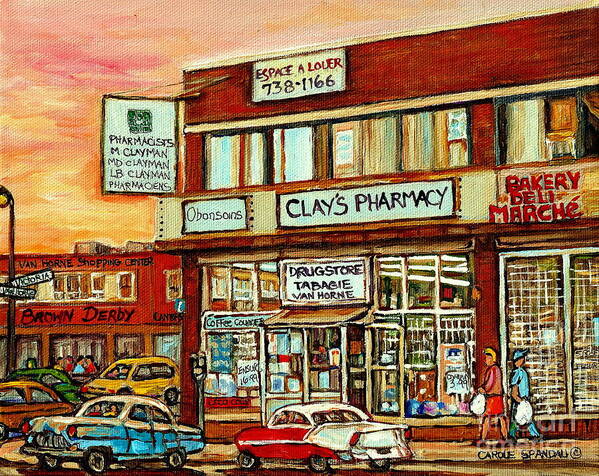The detailed oil painting depicts a vibrant street scene in a 1950s-style business district. The foreground showcases a bustling sidewalk along a colorful red and yellow storefront with various signs. The primary building features signage for "Clay's Pharmacy" and "Drugstore Tabby Van Horn," while an adjacent sign reads "Bakery Deli Maché." Above the pharmacy, a window advertises available commercial space. To the left, another establishment, the "Brown Derby," is prominently displayed. The street is lined with vintage cars, indicative of the 1950s era, along with pedestrians carrying shopping bags. The vivid sky transitions into hues of yellow and pink, adding to the scene's nostalgic charm. In the lower right-hand corner, the painting is credited to Carol Spandu, marked with copyright.